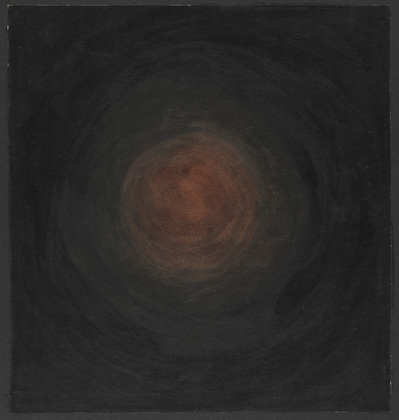The image is an abstract painting, nearly square but slightly taller than it is wide. It predominantly features a grayed-out black background that subtly swirls inward towards the center. The swirling patterns, resembling thick brush strokes or a vortex, reveal a gradation from dark gray to lighter shades as they approach the central focal point. At the heart of the composition, a circular shape with hints of dark orange, brown, and gray emerges, reminiscent of a muted sun obscured by dark clouds. This central area becomes blotchy and less defined with some dark spots, contributing to the overall simplistic yet evocative nature of the painting. The interplay of colors and swirling motion forms a captivating visual effect, creating a sense of depth and movement within the dark and minimalist aesthetic.